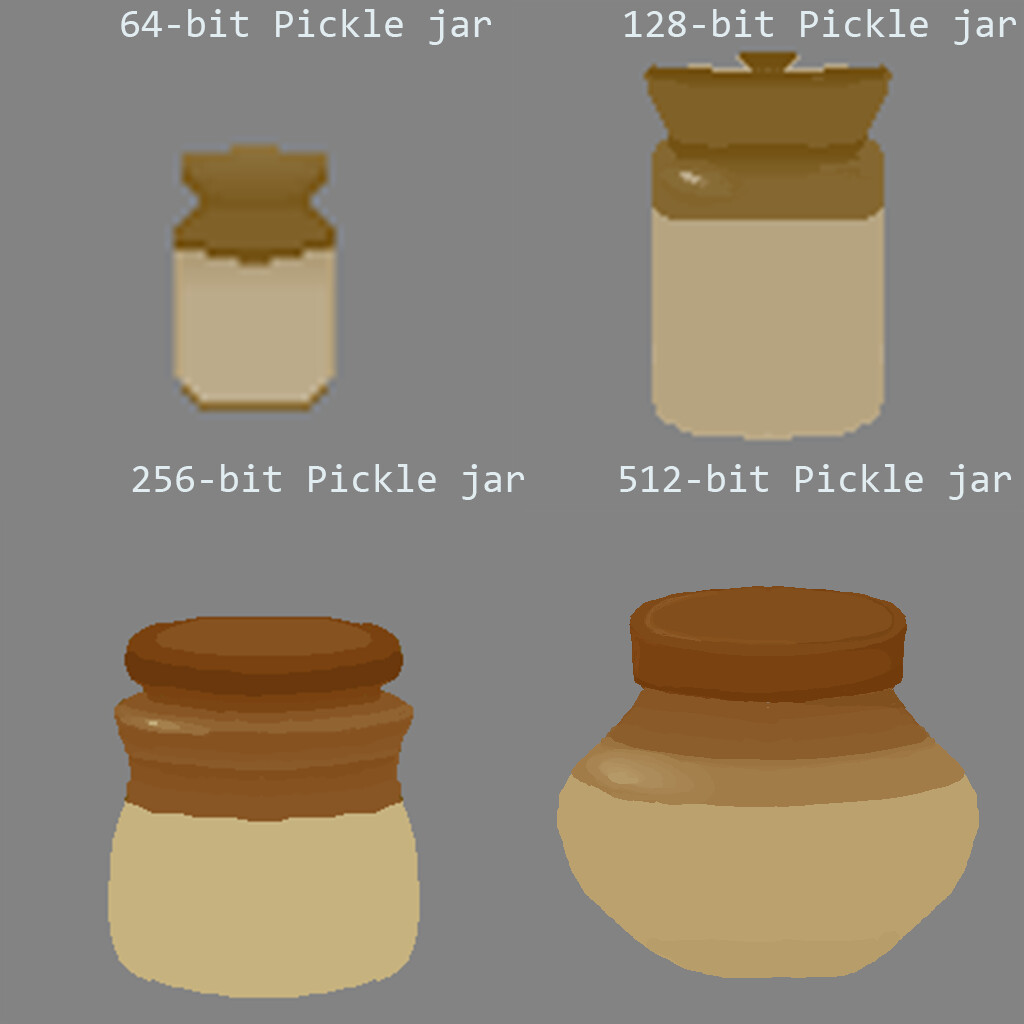This image, crafted with computer graphics, showcases four pickle jars arranged in a 2x2 grid against a gray background. Each jar, increasing in size and bit rate, is labeled with white text: "64-bit pickle jar", "128-bit pickle jar", "256-bit pickle jar", and "512-bit pickle jar". The jars feature varying shades of brown and tan, becoming more finely depicted with higher bit numbers. The 64-bit jar, located at the top left, is the smallest with a light brown body and dark brown neck and cap. To its right, the slightly taller 128-bit jar has a pinkish-tan body and dark brown top. In the bottom left corner, the 256-bit jar is shorter but wider, with a dark brown upper section transitioning to a pinkish-brown body. The largest jar, the 512-bit, on the bottom right, bulges out like a light bulb with a gradient from dark brown at the top to a lighter brown down to the base.